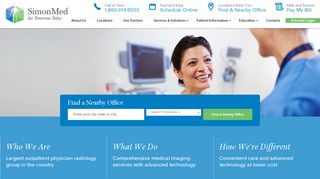The screenshot depicts the homepage of a website named "Simon Med." The site's icon is a three-dimensional cube, with the left half of the cube shaded blue and the right half shaded green, both sides being translucent. In the center of the cube is a white silhouette of a person.

At the top of the page, there's a small blue phone icon labeled "Call or Text" followed by a contact number: 1-866-614-8558. Adjacent to this is a calendar icon that prompts users with "Schedule Online." Further to the right is a location pin icon with the text "Find a Nearby Office," and next to this is an image of a document labeled "Pay My Bill."

Below the header are several navigational links, which include: "About Us," "Location," "Our Business," an unreadable link, "Education," and another unreadable link.

Prominently displayed in the center of the page is a large blue rectangle with the text "Find a Nearby Office." Below this text are fields for users to enter their zip code and other relevant details. Additionally, there is a green box containing information about the organization with the headings: "Who We Are," "What We Do," and "How We're Different."